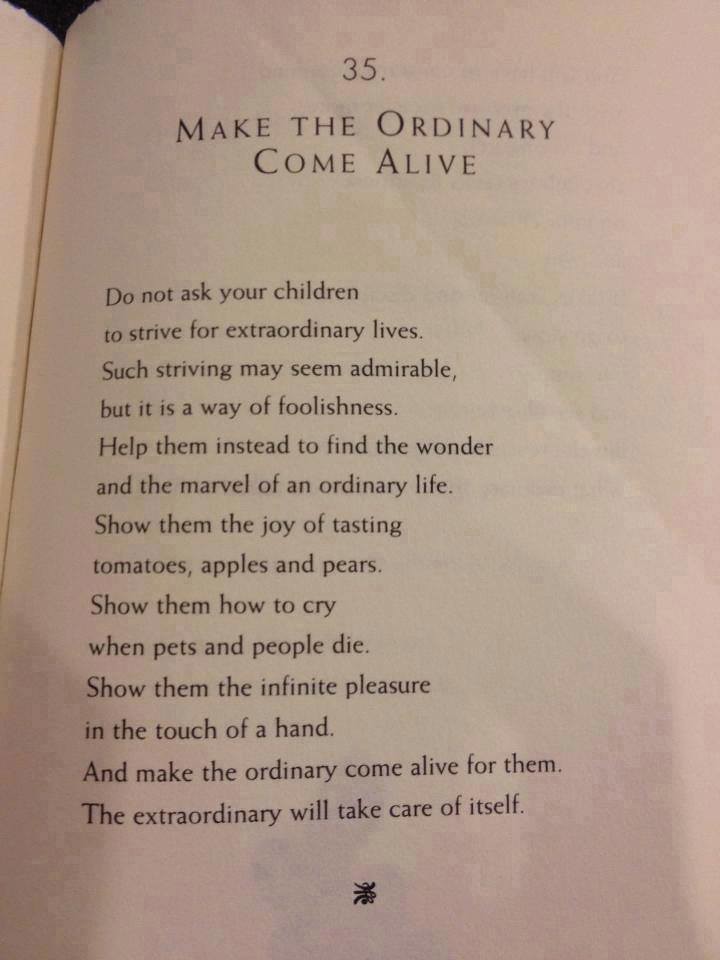This close-up photograph captures a page from a book, focusing on a poem titled "Make the Ordinary Come Alive" prominently labeled with the number 35 at the top. The photograph reveals the crisp white background of the page, accentuating the stark black text. The poem, exuding a self-help essence, advises against urging children to pursue extraordinary lives, suggesting that such aspirations, although seemingly admirable, are ultimately misguided. Instead, it advocates for encouraging children to discover the marvel and wonder within an ordinary life, emphasizing the simple joys of tasting fruits like tomatoes, apples, and pears.